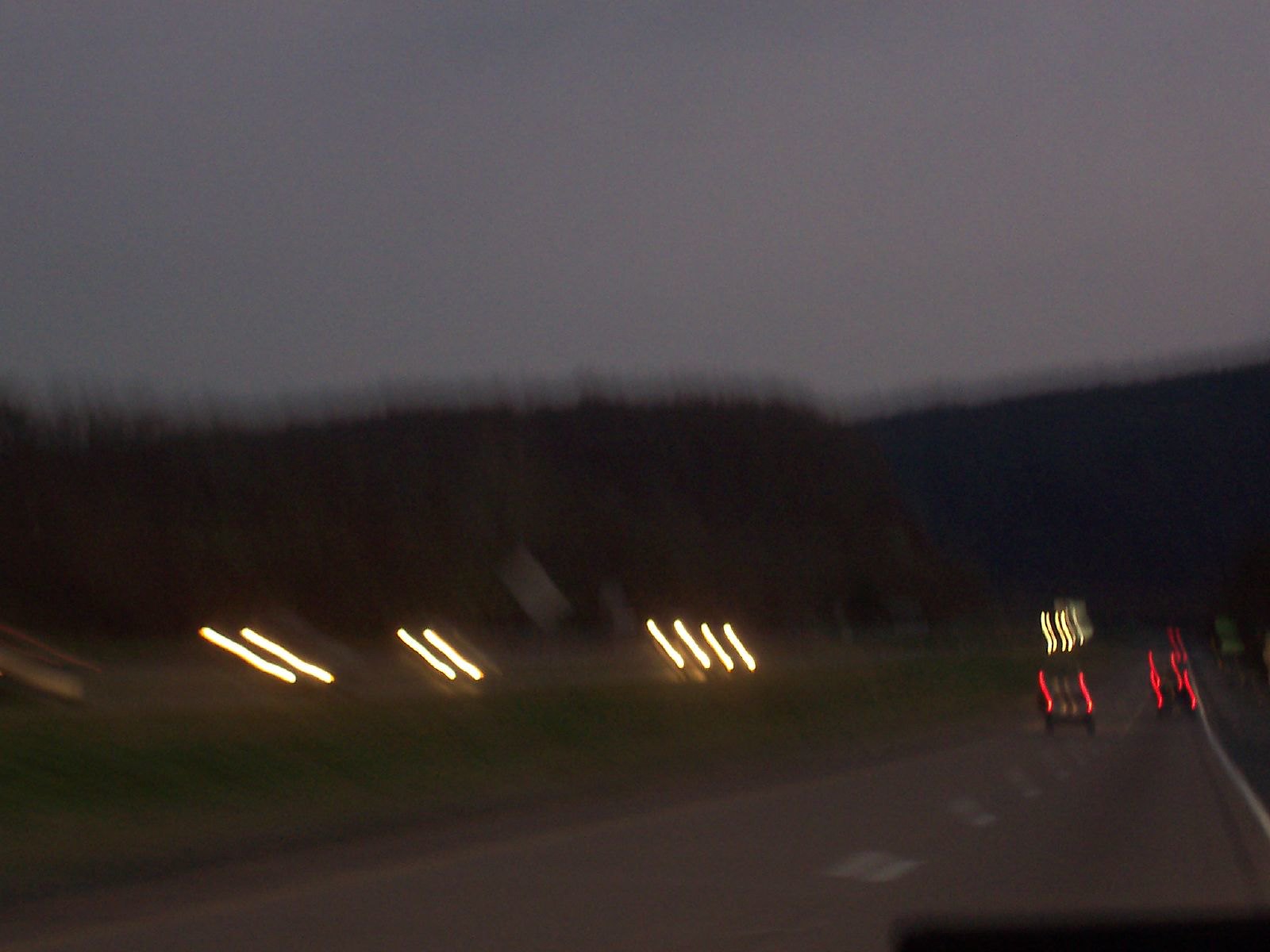A blurry photograph of a bustling four-lane highway at night. On the right side, two lanes are visible, marked by faint white lines, with the red taillights of two cars illuminating the scene. On the left, another set of two lanes is discernible, featuring the scattered glow of five sets of headlights from oncoming vehicles. The sides of the road are vaguely outlined by yellow lines. In the background, dark, indistinct shapes suggest the presence of trees, adding depth to the otherwise indistinct image. The overall blurriness makes it challenging to pick out more details.